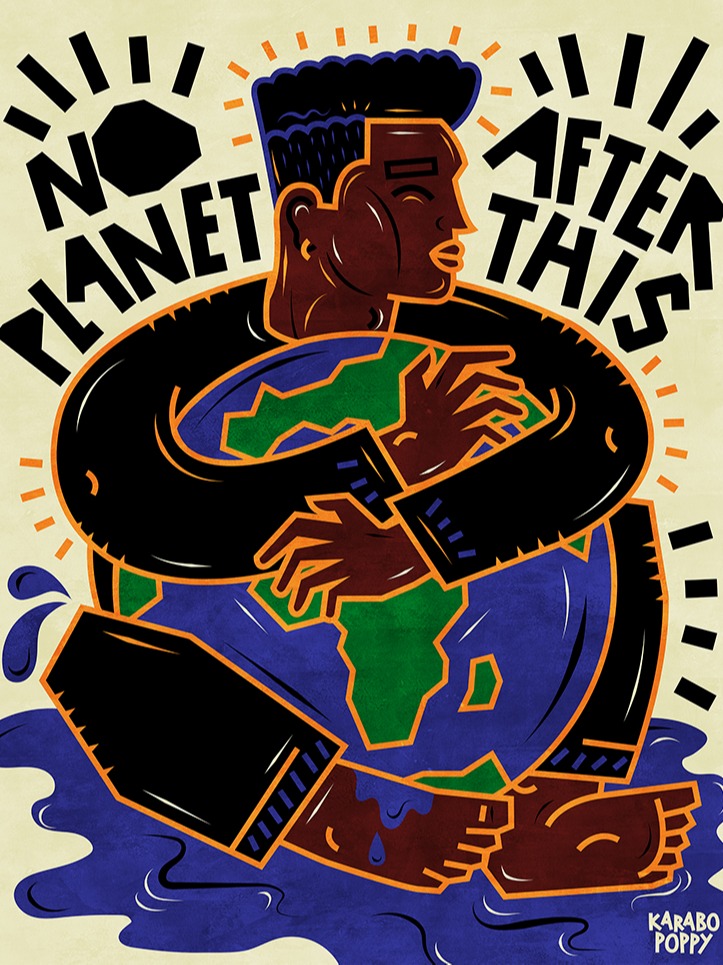This vertical poster features a central illustration of a black man with short hair, dressed in a black outfit, hugging a globe that showcases green continents and blue oceans. The globe is nestled between his crossed legs and his arms as he gently cradles it. Around the globe, it looks like blue water is dripping and pooling beneath, forming splashes around him, giving the impression that he is sitting in a puddle. The background is a light yellowish-cream color. At the top of the image, large artistic block lettering in black reads "No Planet After This," with black sun rays emanating from the text. Additionally, there are orange and black dashes radiating from the man's hair and arms, enhancing the visual intensity. In the bottom right-hand corner, in white writing, it says "Karabu Papi."